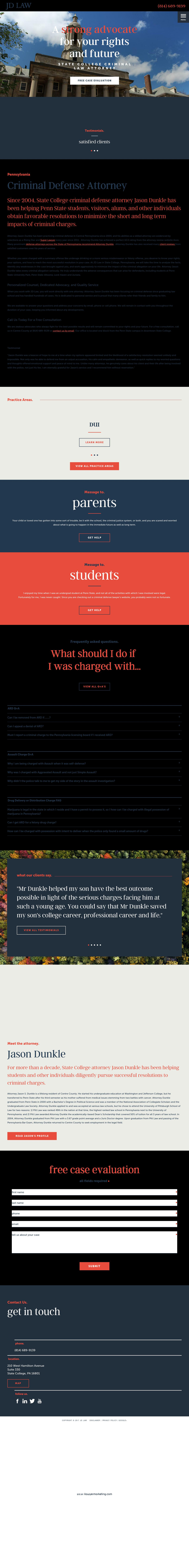The image consists of three stacked screenshots highlighting the services of State College criminal defense attorney, Jason Dunkle. Here’s a more detailed and refined caption for the image:

---

Title: Jason Dunkle - Experienced Criminal Defense Attorney 

Description: 
In the top screenshot, a bold statement reads: "Strong advocate for your rights and future." This is followed by "State College Criminal Law Attorney," emphasizing Jason Dunkle's dedication to criminal defense since 2004. The text elaborates on his extensive experience in helping Penn State students, visitors, alumni, and other individuals secure favorable outcomes in criminal cases to mitigate both immediate and long-term consequences.

Background: An image of an old brick building with classical pillars and a tower stands against a backdrop of blue skies and clouds, symbolizing the prestige and reliability of Mr. Dunkle's law practice.

Proactive Practice Areas: The interface includes clickable options like "DUI," "Learn More," "View All Practice Areas," "Message to Parents," and "Message to Students," providing targeted avenues for assistance and information.

Client Testimonial: The second screenshot features a heartfelt testimonial reading, "Mr. Dunkle helped my son achieve the best possible outcome considering the serious charges he faced at such a young age. You could say that Mr. Dunkle saved my son's college career, professional career, and life," underscoring the profound impact of his legal support.

Experience: The third screenshot reiterates Jason Dunkle’s decade-long commitment to diligently pursuing successful resolutions for his clients, highlighting his extensive experience in criminal defense.

Call to Action: The image includes prompts to "Read Jason's Profile," access a "Free Case Evaluation," and fields to enter contact details, inviting potential clients to take the next step in securing expert legal representation.

---

This detailed caption provides a clear and comprehensive overview of the information presented in the screenshots, emphasizing key points about Jason Dunkle's expertise, client success stories, and available resources for support.